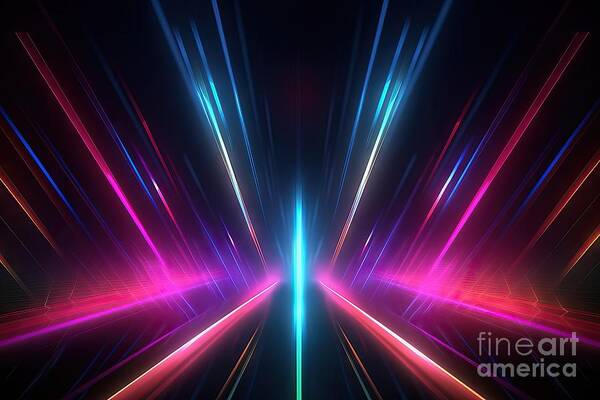The image depicts an array of vibrant, colorful light streams set against a dark, almost black background. These streams include hues of magenta, blue, green, and dark purple, creating a striking contrast. Originating from the bottom middle of the image, the light streams fan outwards in various directions toward the top corners and sides. Prominent red and blue lines stretch upward, becoming more luminescent as they approach the center, while thinner orange and gray lines accompany them. The top of the image features additional blue, red, and pink lights that converge towards the center. The bottom right corner bears a watermark that reads "Fine Art America," with the word "art" bolded and the text in a sans serif font. The vibrant colors and dynamic arrangement grant the image a festive and lively atmosphere.